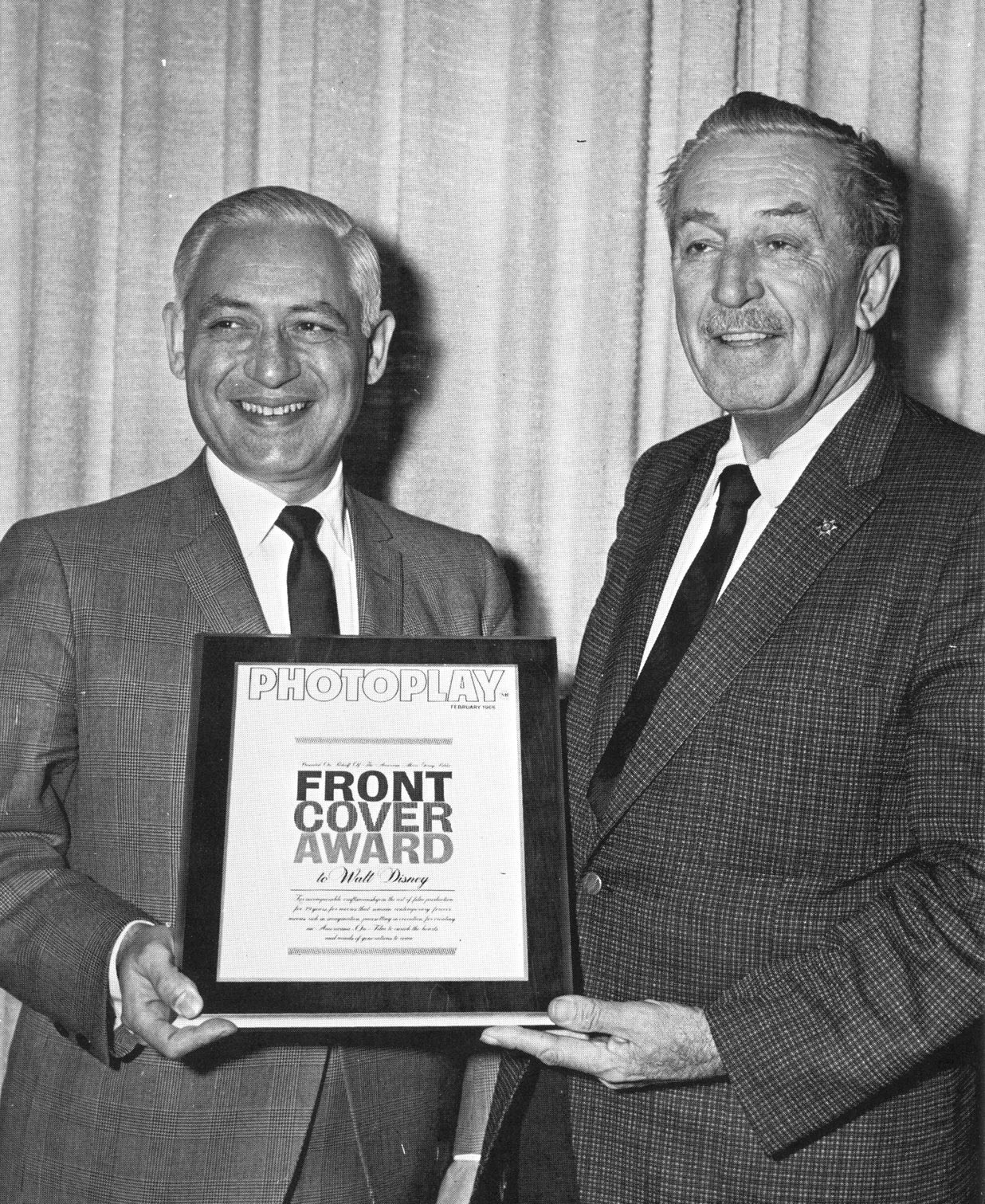The black-and-white photograph captures two older, smiling gentlemen standing side by side in front of a light-colored, slightly folded curtain. Both men are dressed in business suits with black ties and collared shirts, their jackets slightly open. The man on the right, who appears significantly older, sports a checkered plaid shirt with a central button and outstretches a slightly hairy hand to hold the award. Both have short, slicked-back hair styled with gel, aligning with fashion trends of the 1960s or 1970s. They jointly hold a framed plaque inscribed with "Photo Play Front Cover Award," signed by Walt Disney. Although the smaller writing below is unreadable, the award signifies a notable achievement. The scene, likely set during an award ceremony or a news event, features the men smiling and looking into the distance, creating an image of shared accomplishment. The photograph exudes a formal yet celebratory atmosphere, suitable for a newspaper feature or historical documentation.